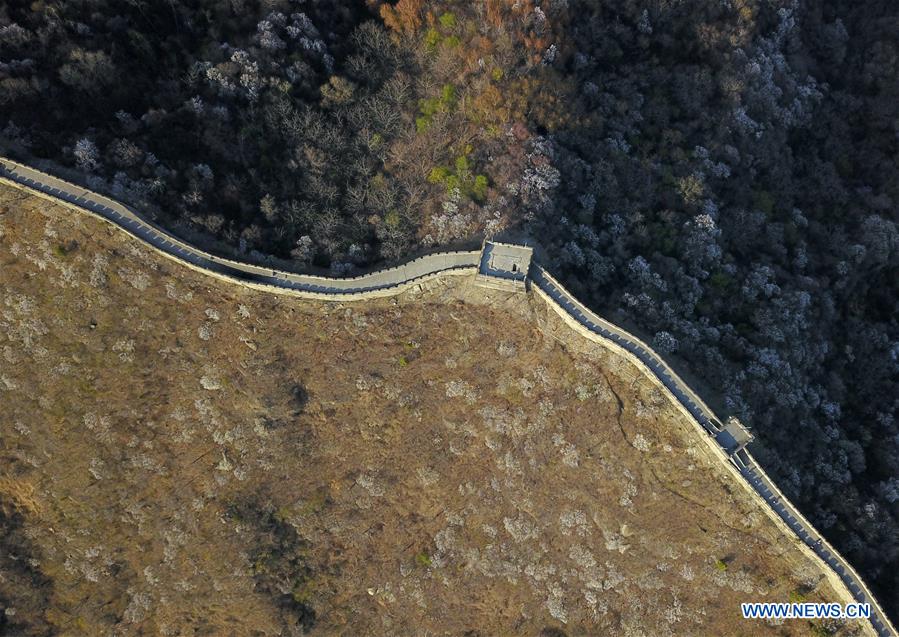This aerial image, likely captured by a drone, presents an expansive overhead view reminiscent of the Great Wall of China. Dominating the center of the image is a long, stone wall with several blocky structures or forts dotting its path, presumably serving as watchtowers or guard posts. The wall itself is constructed along the ridge of a mountainous terrain. To the south of the wall, the landscape appears arid and sparse, characterized by brown grass and desert-like shrubs. In contrast, north of the wall, the terrain is more verdant and diverse, showcasing a dense mixture of trees in varying hues of green, yellow, and brown. Additionally, the trees on the periphery of the image, especially to the left and right, are darker, appearing shadowed or perhaps just naturally denser. The vantage point of the shot is high enough that fine details are minimal, but a small speck, possibly a person on the wall, and a website watermark (news.cn) can be noted in the bottom corner of the image.